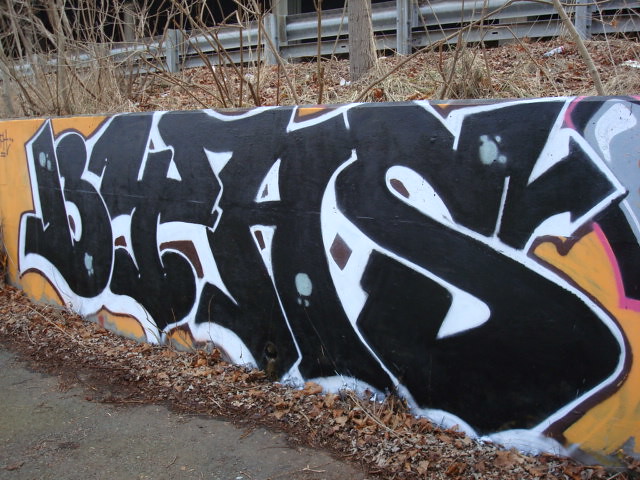In the outdoor winter scene, a photograph depicts the side of a highway bordered by a guardrail at the top. Below the guardrail, there's an embankment covered in brown, dead grass and a scattering of dry leaves intermixed with trash. On the other side of a narrow walkway lies a stone wall, approximately three feet tall, decorated with graffiti. The graffiti features a mix of black, white, yellow, and a hint of pink, though the design is largely unintelligible, appearing as a combination of letters, numbers, and symbols, starting with what looks like an upside-down '1' and the numeral '3', followed by indecipherable characters. The vibrant graffiti contrasts sharply against the dull, brown foliage and the cold, stark surroundings, indicating the harshness of the winter season. Above this scene, the steel guardrail acts as a barrier to prevent cars from veering off the roadway, while bare, leafless trees loom in the background, adding to the overall desolate atmosphere.